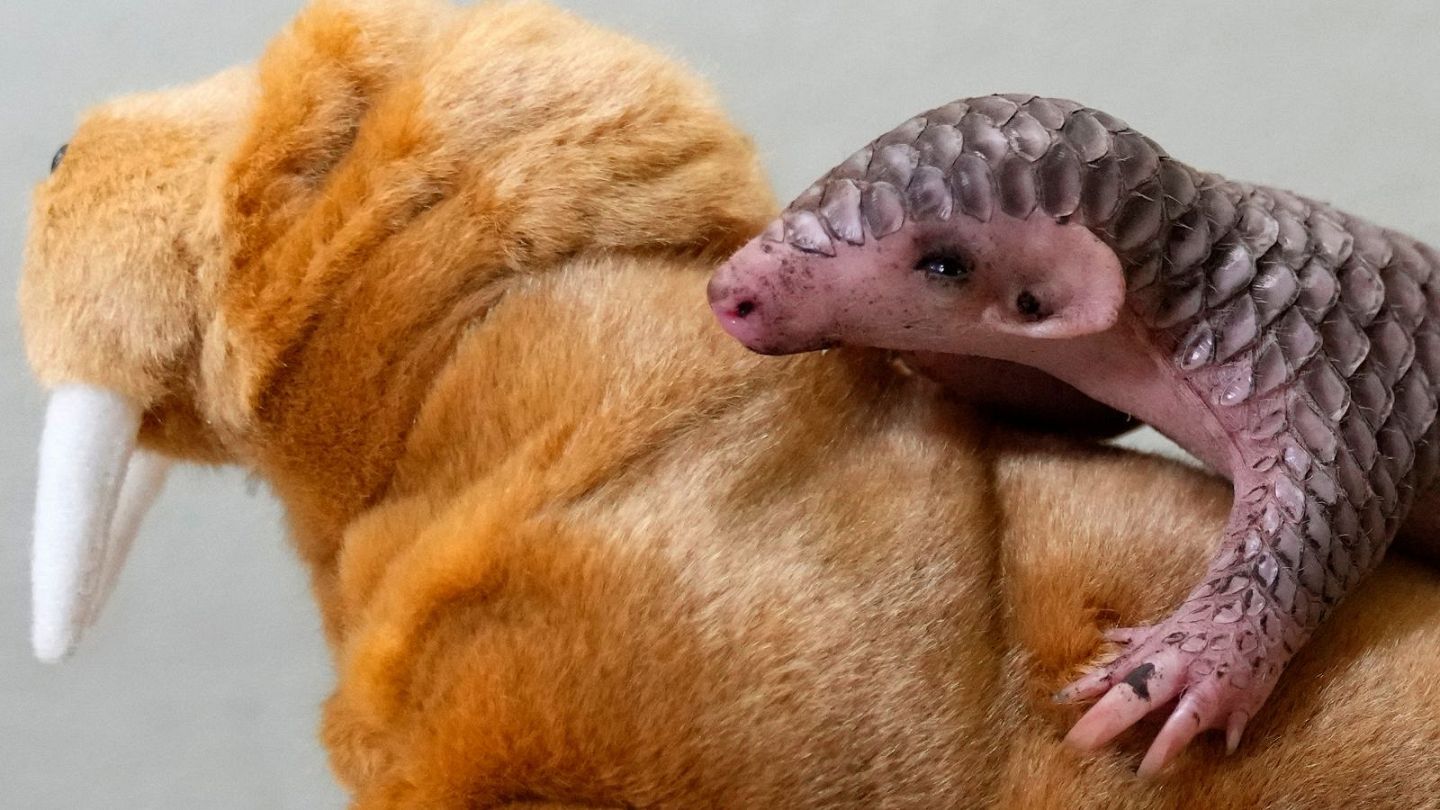In this close-up photograph, a baby armadillo, with a light pink face and pink ears, is perched on the back of a stuffed walrus. The walrus, facing to the left, features a thick, fluffy reddish-brown fur with yellowish tan shadings and prominent white tusks extending from its mouth. Its left tusk is fully visible, while the right tusk is partially obscured. The armadillo's hard, scaly shell and top half of its body display a gradient from light brown to grayish hues, contrasting with its pinkish nose and clawed paw resting on the walrus's back. The background is a pristine white, emphasizing the details and colors of the two figures.